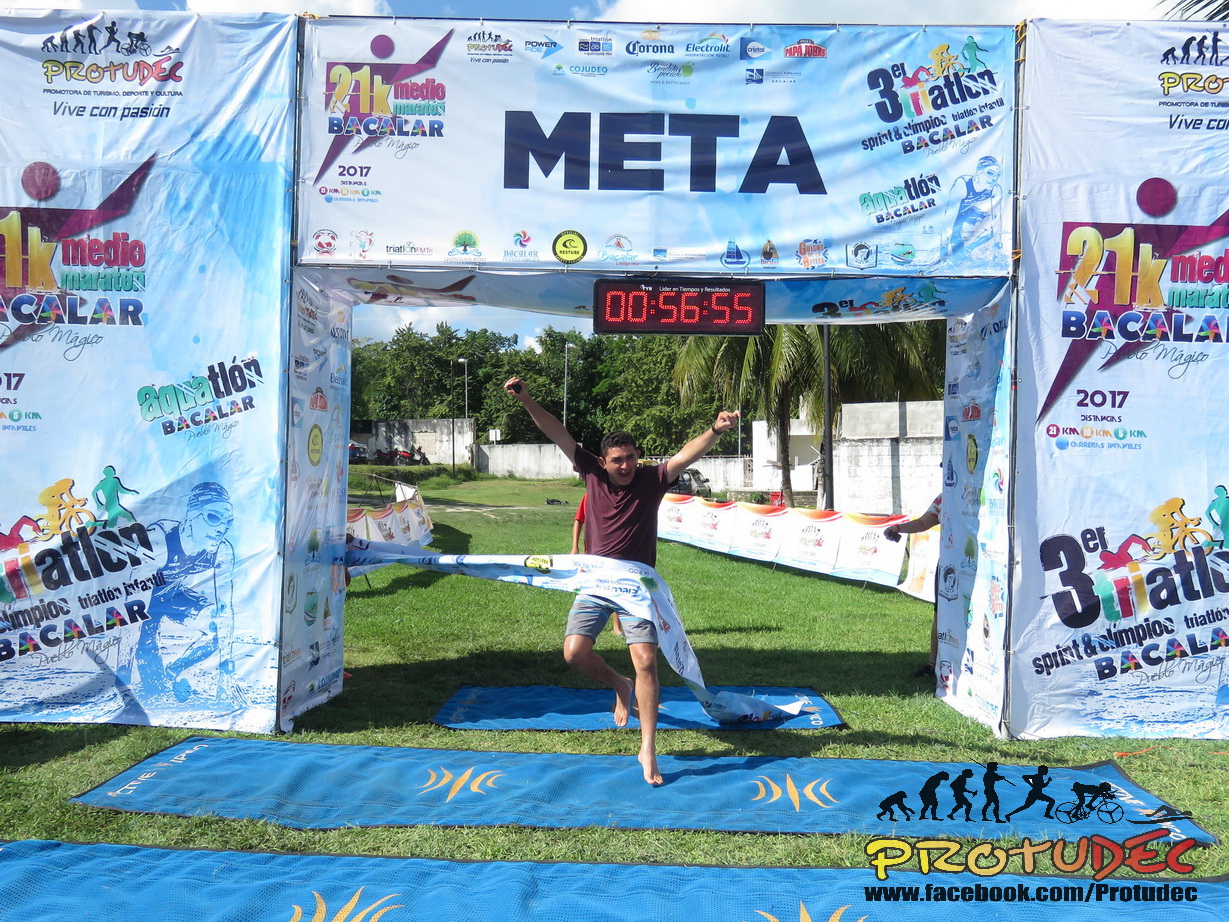A jubilant, barefoot young man is captured crossing the finish line of what appears to be a triathlon event. He has both arms raised in victory, smiling and laughing exuberantly. He is running across a white banner spread between two columns, which marks the finish line. Just beyond the finish line, there is a blue towel and two longer blue towels or rugs laid out for the runners. 

Above him, an electronic clock displays a time of 56 minutes and 55 seconds, while a prominent banner with "M-E-T-A" stretches across the top, hinting at the event's concluding point. The entire area is adorned with banners and images depicting various stages of human evolution, from ape to runner, cyclist, and swimmer, symbolizing the diverse athletic feats involved in the event. 

This triathlon, organized by a company called Protudec, features corporate sponsorship from entities like Aquatlan Bacalar and showcases its logo prominently. The event appears to take place in the early evening, with the contestant trailing behind him also barefoot, raising questions about the formality of their participation. Despite the ambiguous nature of the competition, the scene exudes a sense of triumph and joyous achievement.